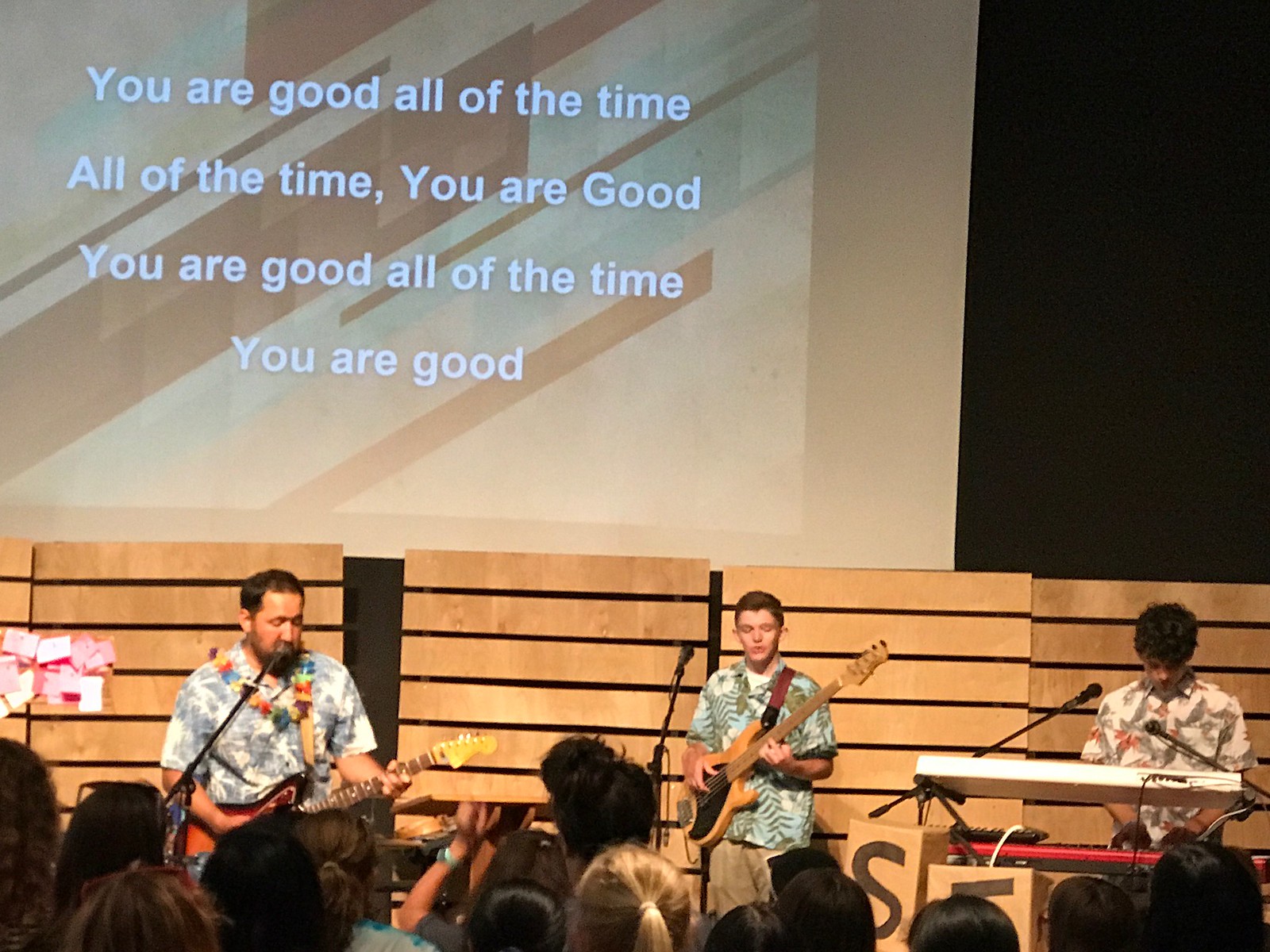A small band of three musicians stands on a wooden stage, each donning button-down collared shirts with vibrant floral designs, reminiscent of Hawaiian themes. On the far left, a man with a colorful rainbow flower lei around his neck sings into a microphone while playing a brown, black, and yellow electric guitar. He wears a distinctive shirt with flowers printed on it. Standing next to him, at the center of the stage, is another man also dressed in a button-down floral shirt. He strums a brown and black electric guitar and stands in front of a microphone. On the far right, a keyboardist with curly hair looks down at his lower red keyboard, with a white keyboard placed higher in front of him. His shirt, adorned with larger floral prints of gray, light rose, and white hues, complements the group's vibrant appearance. The stage features a wooden panel wall as a backdrop, behind which words are displayed: "You are good all of the time, all of the time you are good," suggesting that the lyrics of the song are printed for audience participation.